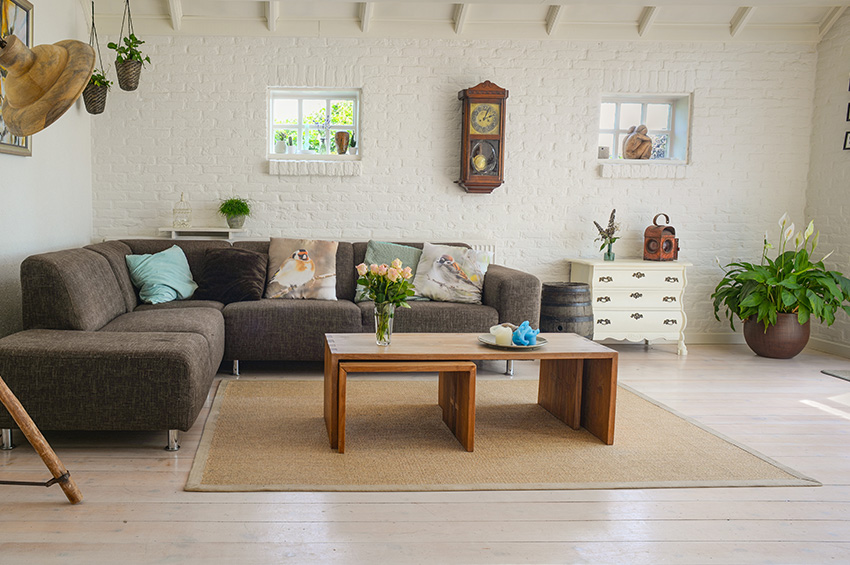This detailed description captures the essence of a cozy, well-decorated living room, which appears to be either a home or an apartment and resembles a 3D color elevation rendering, possibly created using an app like SketchUp. The room features white painted brick walls and a beige wood-paneled floor, complemented by a deep beige square rug. Central to the room is an L-shaped, armless sectional sofa adorned with a variety of throw pillows in aqua, black, turquoise, and beige tones, including some pillows with bird designs.

In front of the sectional is a light wood nested coffee table, supporting a clear glass vase with peach-colored roses and a gray plate with a candle. To the right of the sofa, a white three-drawer credenza holds additional decorative items. A large bronze planter in the far-right corner bursts with green and white ferns spilling over its sides and white lily-shaped flowers towering above.

The back wall features a wall clock with a light brown wooden frame and a pendulum encased in a small glass compartment, positioned between two windows. Each window consists of six glass panes in a white frame and sits above a small brick ledge. In one window, a statue stands, while the other hosts a base, together adding a personal touch. Hanging plants dangle from the ceiling, contributing to the room's verdant feel. Exposed white-painted beams along the ceiling and a brass-colored light fixture facing the sofa complete the serene, stylish ambiance of this imagined space.